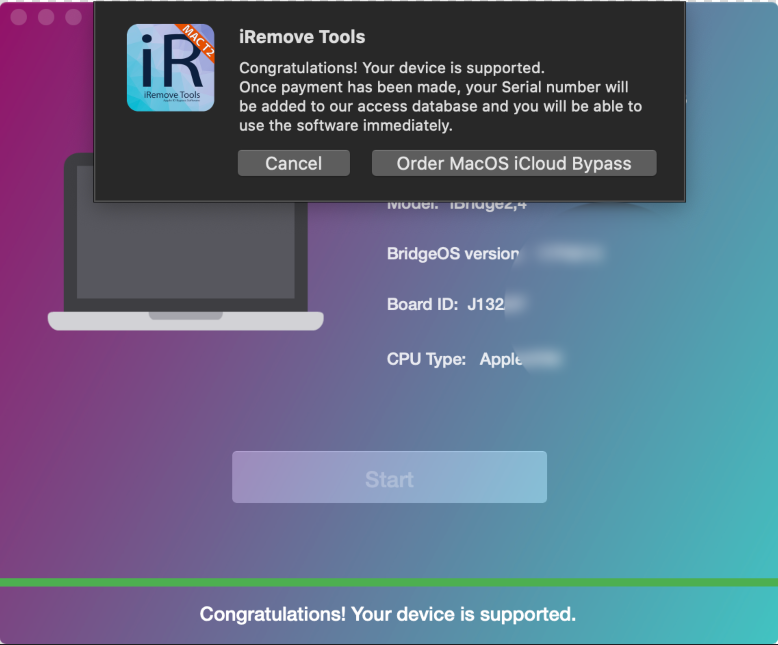The image showcases a colorful, gradient background starting from the left with pink, transitioning to purple, followed by a grayish hue, and finally turning green on the right-hand side. Centrally located at the top is a black, rectangular pop-up window. In the pop-up's upper left corner, there is a blue and gray icon with the letters "IR" in dark text, alongside a diagonal orange banner that reads "Mac" in white. To the right of this icon, on the black background, are white letters that state, "I remove tools. Congratulations, your device is supported."

At the bottom of the pop-up window are two rectangular gray buttons; the left one is labeled "Cancel" in white text, and the right one says "Order macOS iCloud bypass." Below this black window and to the left, there is a cartoonish icon resembling a computer monitor attached to a gray laptop base. Beneath the black pop-up window to the right are lines of white text which start clearly but become increasingly blurred towards the right edge of the image. The partially readable text includes, "Bridge OS version," followed by "Board ID: J132," and "CPU type: APPLE," with the remainder of the lines blurred out.

At the bottom of the image is another gray rectangular button labeled "Start," which is grayed out. A vivid green horizontal line spans across the very bottom, underneath which the bolded white text states, "Congratulations, your device is supported."